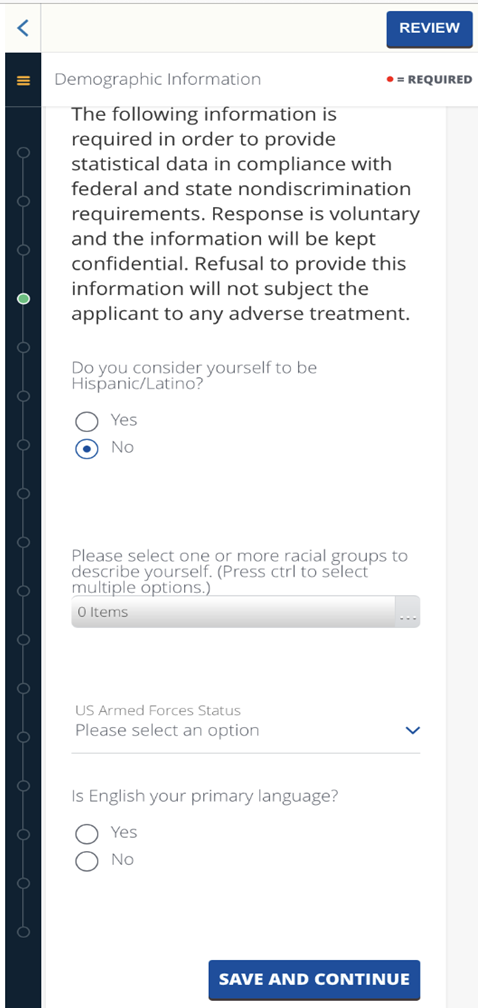In the image, the top right corner features a blue button labeled "Review." On the bottom left, the text "Demographic Information" is displayed, accompanied by a red dot indicating that the information is "Required." 

Centrally located on the page, the text explains, "The following information is required in order to provide statistical data in compliance with federal and state non-discrimination requirements. Response is voluntary, and the information will be kept confidential. Refusal to provide this information will not subject the applicant to any adverse treatment."

Further down, a question asks, "Do you consider yourself to be Hispanic or Latino?" with circular checkboxes labeled "Yes" and "No." In this instance, "No" is highlighted in blue.

Below this, the text prompts, "Please select one or more racial groups to describe yourself. Press Ctrl to select multiple options." A drop-down menu is present underneath, noting "0 items."

Following this is a section titled "U.S. Armed Forces Status," with instructions to select an option from another drop-down menu.

Subsequently, the page inquires, "Is English your primary language?" with two checkboxes for "Yes" and "No."

Finally, at the bottom right, a blue button with white text reads "Save and Continue."